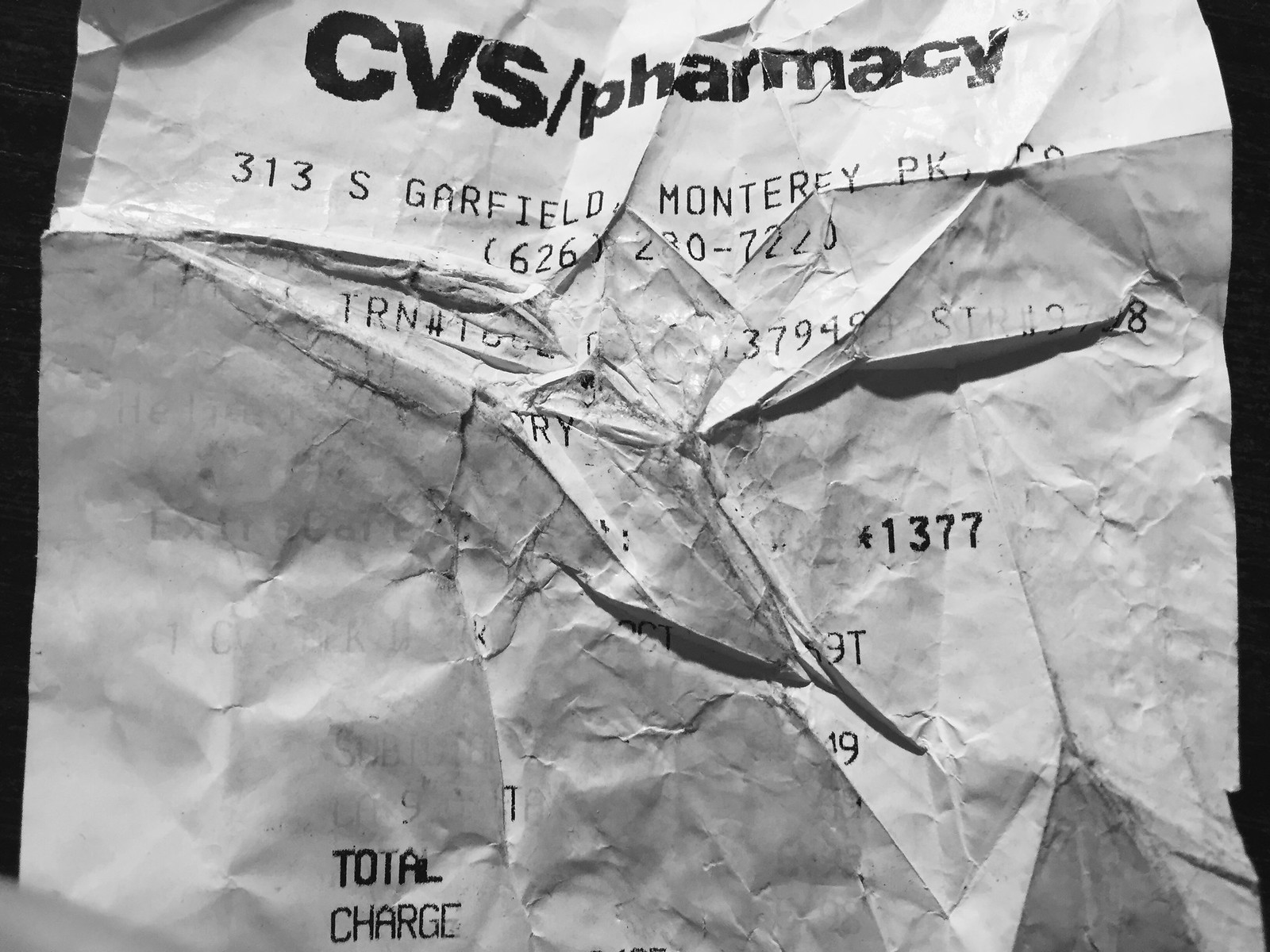This is a close-up photograph of a highly crumpled and faded CVS Pharmacy receipt. The receipt, likely a discarded piece of trash, is taken in black and white, showcasing various shades of white and gray with black lettering. The CVS Pharmacy logo is prominently displayed at the top, followed by the address “313 South Garfield, Monterey Park,” with the state uncertain due to smudging—either California or Colorado. A partially visible phone number, "626-280-7220," is listed beneath the address. The surface of the receipt is rough, characterized by extensive wrinkles, which have rendered most of the text illegible or erased. Despite these distortions, "Total Charge" can be seen in the lower left corner alongside the fragmentary number “1377” midway down on the right. The image captures the receipt against a thin strip of black background on either side, framing the crumpled document as its central focus.